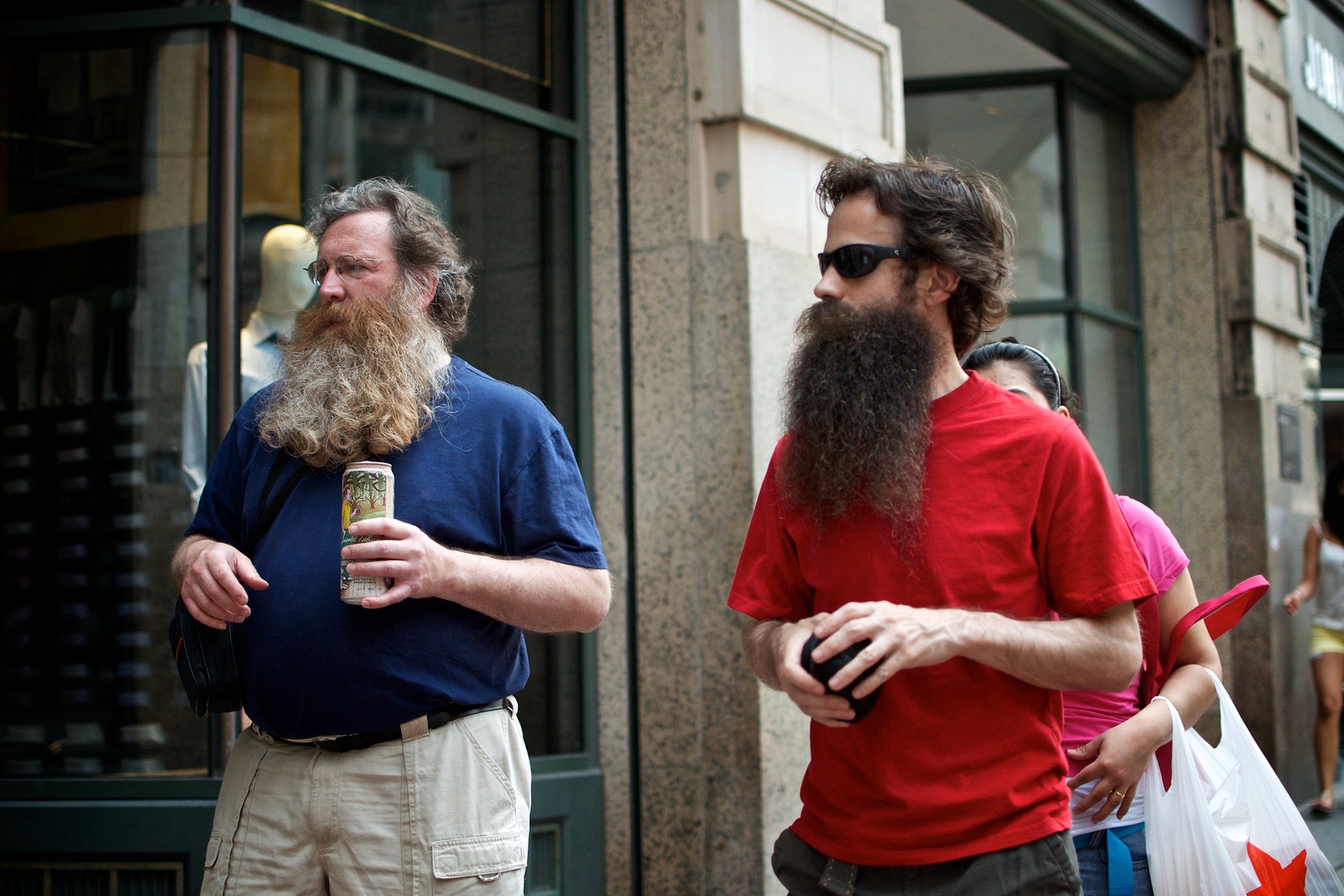In a rectangular outdoor photograph, three individuals are depicted walking along a sidewalk adjacent to a series of stores. Prominent among them are two bearded men. The older gentleman on the left, reminiscent of Santa Claus with his long white beard, sports a blue t-shirt, khaki cargo shorts, and a pair of glasses. Slung over his shoulder is a black satchel, and he holds a tall beverage can in one hand. Walking beside him is a younger man with a dark, extensive beard and brown hair, probably in his thirties. He’s attired in a red t-shirt, dark sunglasses, and dark khaki shorts, holding what seems to be either a small wallet or a cell phone. Just behind them appears a shorter woman with dark hair pulled back with a headband. She’s wearing a bright pink t-shirt and carrying a white plastic shopping bag, which has a red star on it. The background showcases store windows, with one distinct window to the left featuring a mannequin dressed in a blue shirt.